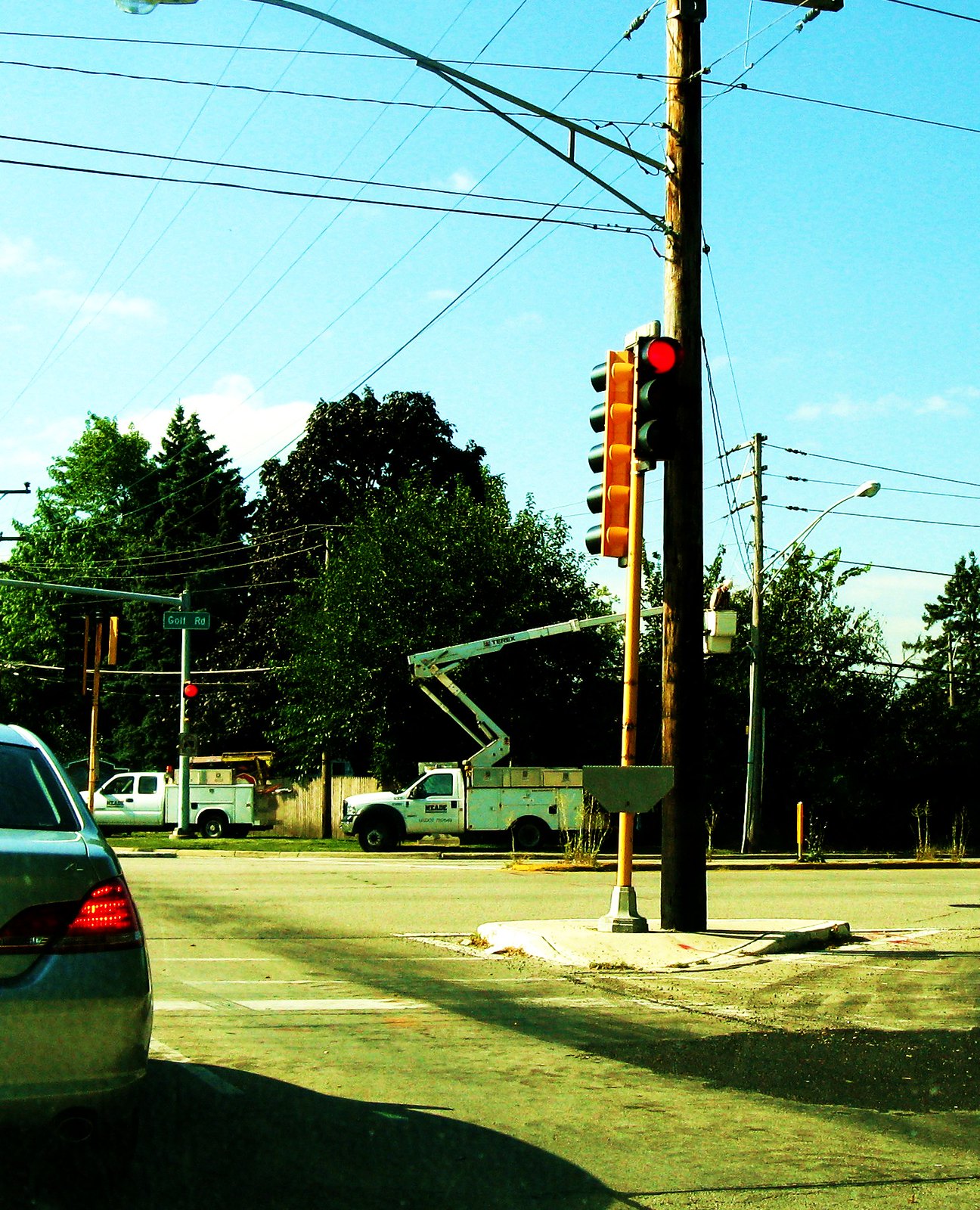The photograph captures a sunny outdoor daytime scene with a vivid blue sky scattered with white clouds. In the background, there's a dense line of green trees beneath the clear sky. The scene is set at an intersection notable for its busy network of telephone poles and electric wires crisscrossing the area. Prominently, a tall yellow metal pole equipped with a traffic light shows a red signal, while wires stretch in various directions from multiple utility poles. 

In the foreground, there is a blue car halted at the crosswalk, its red taillight illuminated. The intersection appears shaded, giving the roads a mossy green appearance despite the bright day. Dominating the right side, two work trucks, painted in greenish turquoise, are parked along the street. The foremost truck has a ladder stowed on its back, whereas the truck behind it has its ladder raised, indicating a worker is positioned to conduct repairs on the utility wires. The detailed composition reveals a typical busy street scene with utility maintenance, framed by the sunlit sky.